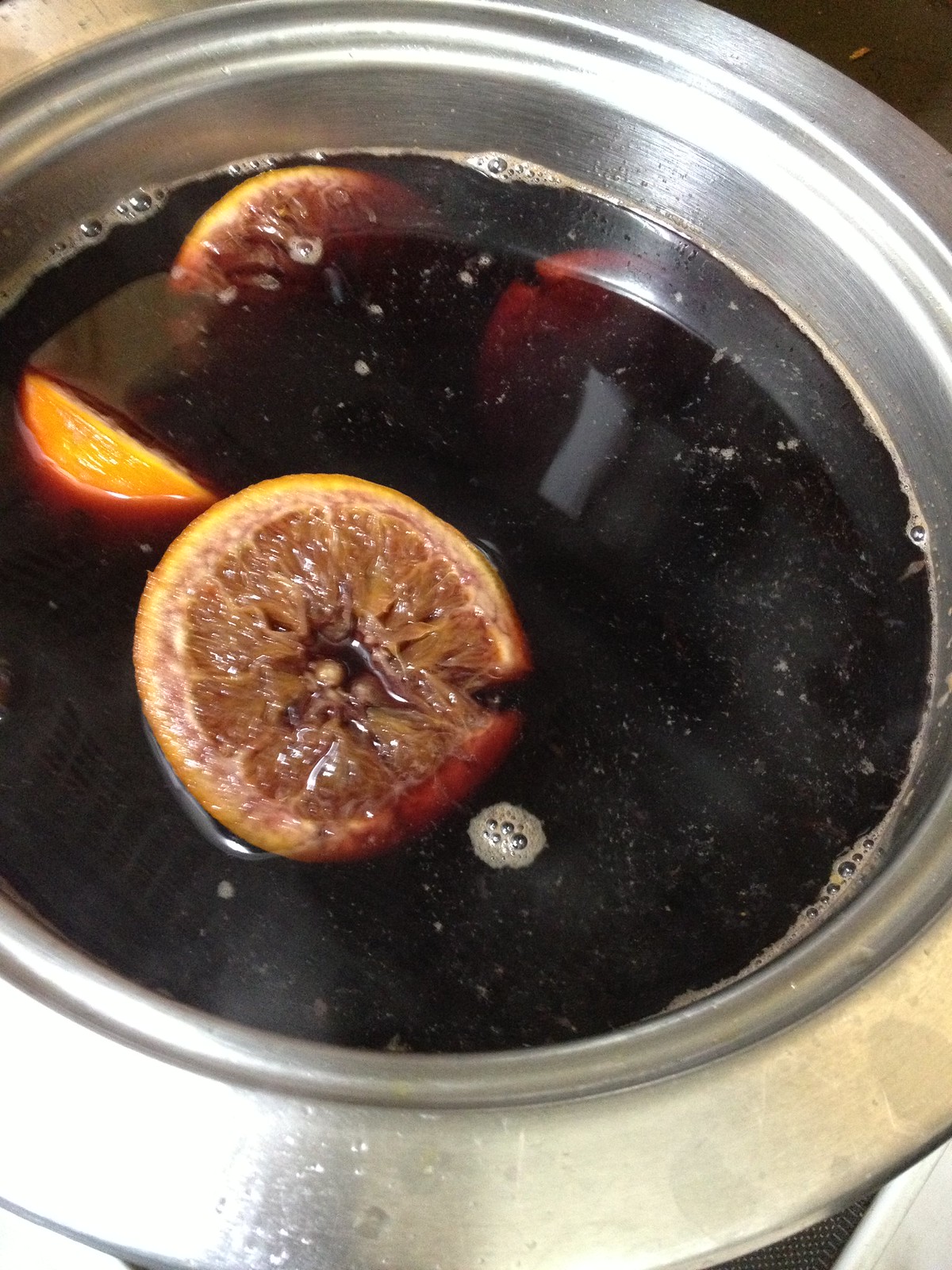The image depicts a metal container, possibly a bowl or pan, filled with a murky, dark liquid that appears almost black. Floating within this liquid are segments of a citrus fruit, likely grapefruit or orange, which look old, musty, and unappetizing. The fruit appears to be cut into pieces, with at least three sections visible. The liquid has bubbles along the edge, suggesting it could be some form of broth or herbal concoction. The setting is likely indoors, indicated by the reflection of overhead lighting on the container. The overall scene is quite unappealing, characterized by a mix of dark liquid and deteriorating fruit, creating an impression of something poorly prepared or left to spoil.